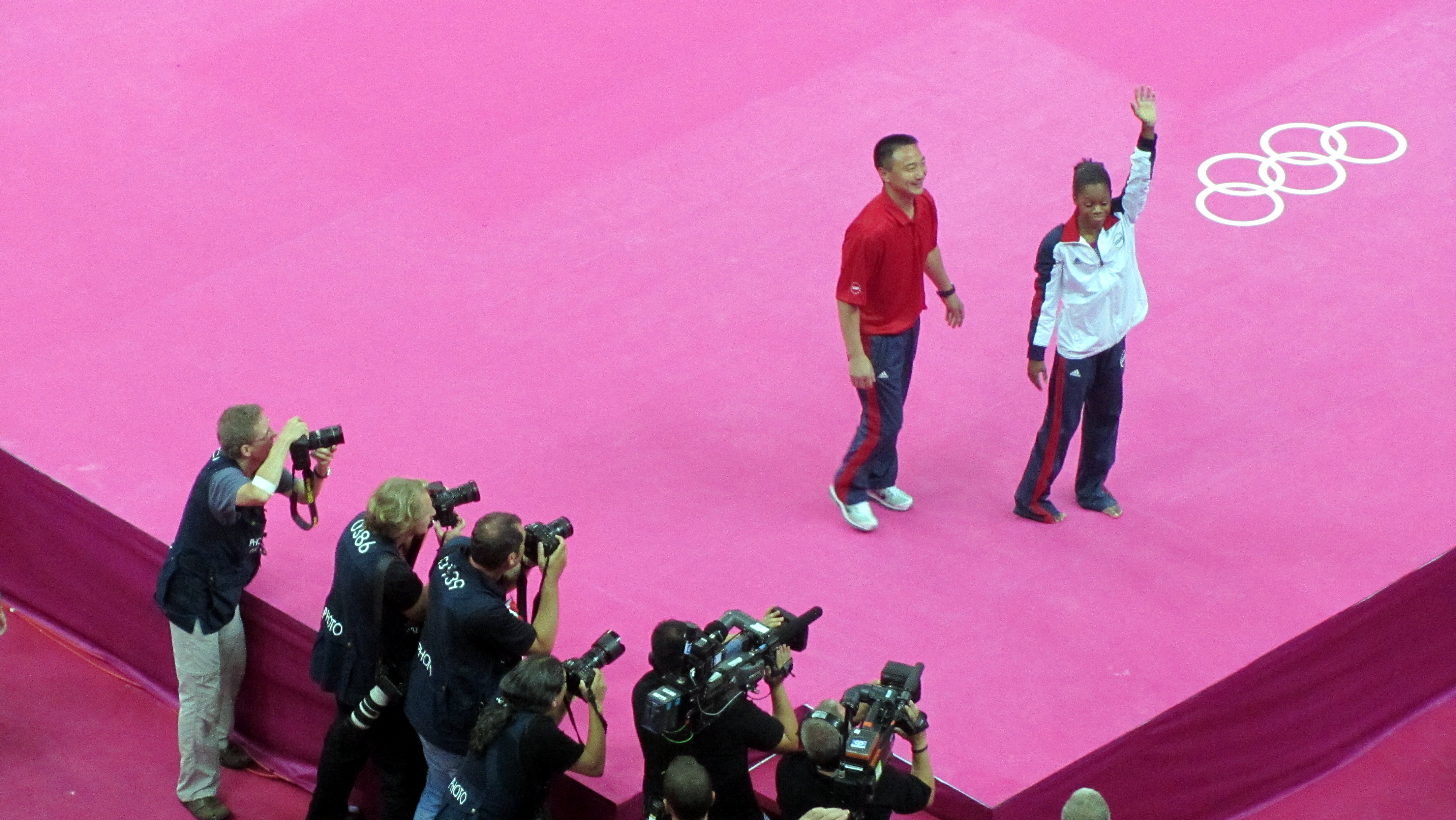The photograph captures a vibrant moment at an Olympic gymnastics event from an elevated perspective. Dominating the right-hand side of the image is a young woman, likely an American gymnast, distinguished by her red, white, and blue jacket, and dark blue pants with a red stripe down the leg. She has black hair tied back and holds her left hand high in the air, facing slightly to the right. Beside her and a bit behind stands a man, presumably her coach, with short black hair. He wears a red short-sleeved shirt, matching blue pants with a red stripe, white shoes, and a watch on his left wrist. Both figures are situated on a large pink platform, adorned with the iconic white Olympic rings towards the right and slightly behind them, suggesting they are on gymnastic floor exercise apparatus often used in Olympic settings. Surrounding the platform is a maroon edge, partly visible at the bottom of the image. Gathered around the corner of the platform, several photographers in black shirts focus their cameras forward, capturing the action, while two of them wield larger camcorders aimed at the gymnast and her coach.